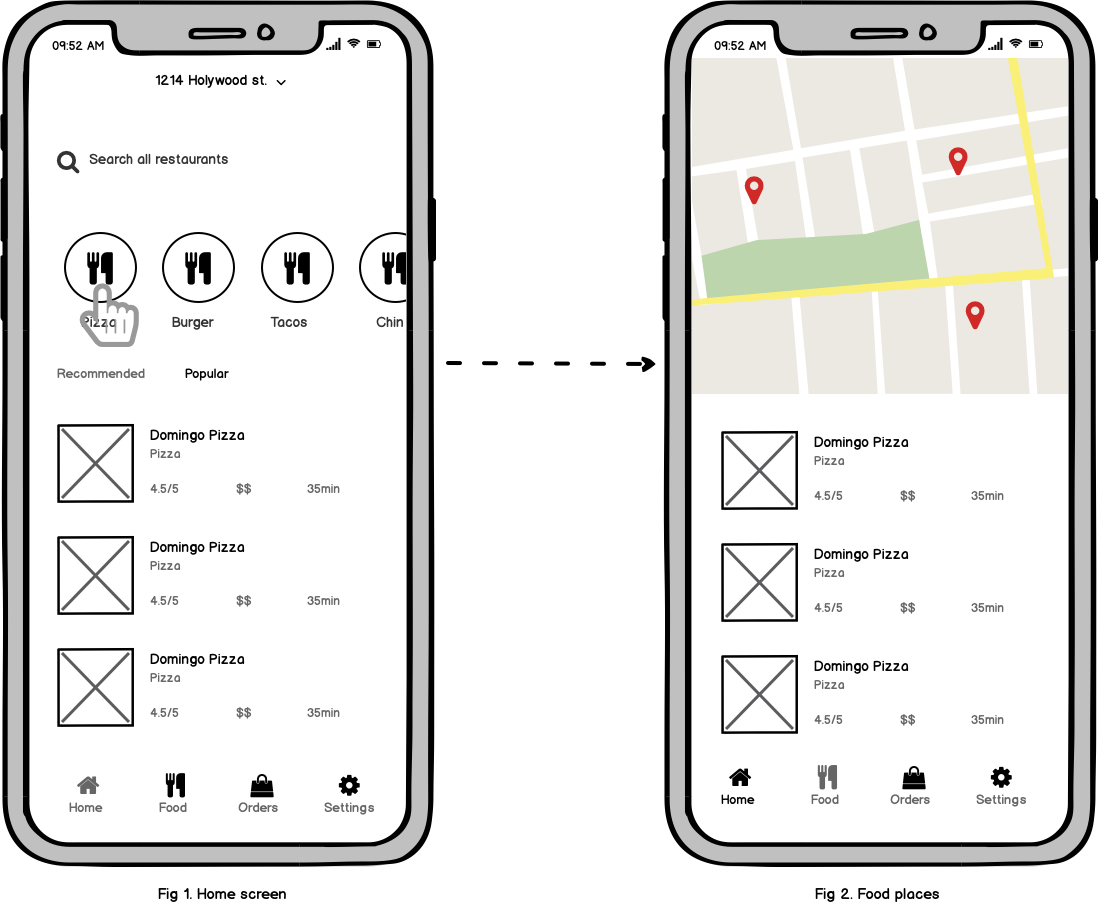This black and white illustration depicts two vertically-aligned, rectangular cell phone screens encased in thick gray borders. Beneath the screens, the left one is labeled "Figure 1: Home Screen" and the right one "Figure 2: Food Places." A dashed black arrow points from Figure 1 to Figure 2, indicating a transition between the screens.

The left screen, Figure 1, displays a food delivery app interface. At the very top, the time is shown as 9:52 a.m. and the location as 12 14 Hollywood Street. A search bar reads "Search all restaurants." Below it, there are four circular icons labeled "Pizza," "Burger," "Tacos," and "Chinese," with a gray finger hovering over the "Pizza" button. The area beneath showcases three identical listings for "Domingo Pizza," all rated 4.5 out of 5 stars, costing two dollar signs ($$), and each 35 minutes away. Icons at the bottom of the screen provide quick access to "Home," "Food," "Orders," and "Settings."

The right screen, Figure 2, represents the detailed screen for selected pizza places. Its top half features a map with three red teardrop-shaped markers indicating the locations of Domingo Pizza. Below the map, the same listing for Domingo Pizza appears three times, maintaining the same star rating and estimated delivery time of 35 minutes.

This illustration effectively demonstrates the user’s progression from a general food search screen to a specific pizza place locations screen within the app.